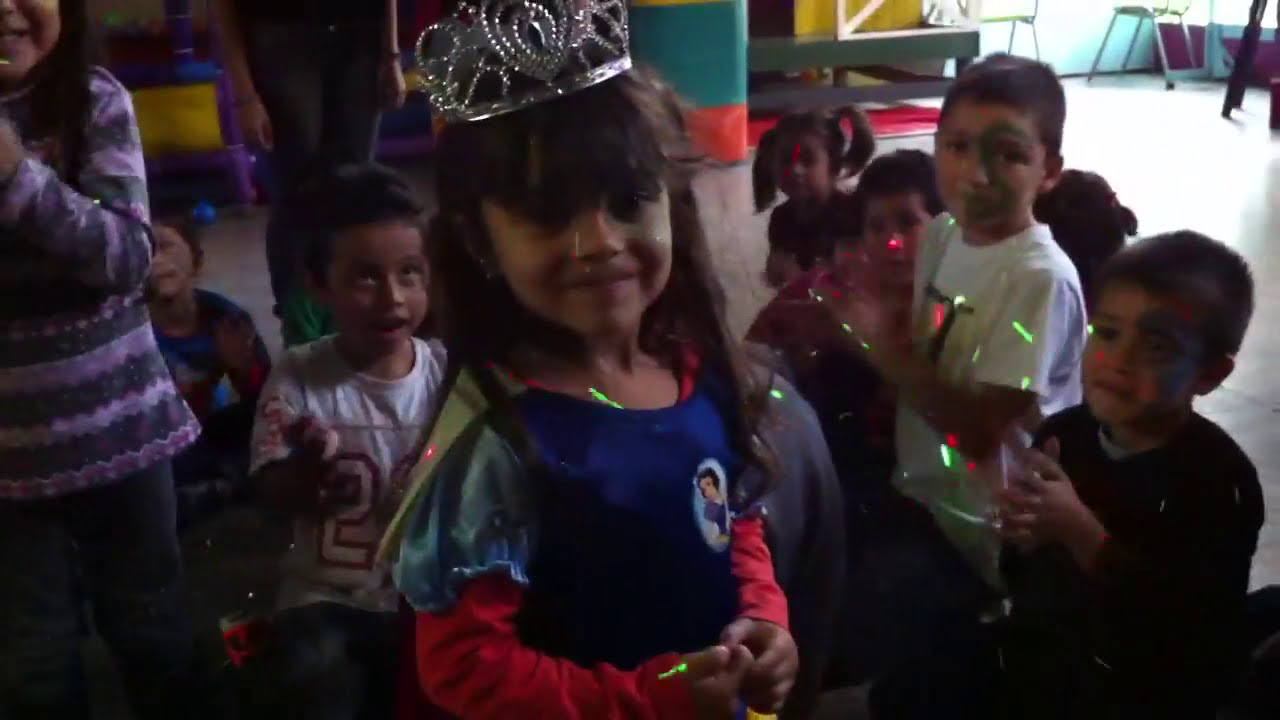A cheerful scene unfolds indoors where a group of small children is gathered. In the center stands a young girl wearing a silver crown, with her long brunette hair cascading just above her eyes and down to her shoulders. She is dressed in a Snow White princess costume, featuring a white chest, red sleeves, and a patch of Sleeping Beauty. Surrounding her are various children illuminated by green and red strobe lights. Directly behind her on the left side, there is a shorter child in a white jersey with the number two, gazing upwards. On the right is another cluster of kids, with the tallest boy dressed in a white shirt, sporting black hair and green face paint. To the far right stands a shorter child with closely cropped hair, wearing a black shirt and clasping his hands together, with red paint on his face. Additionally, behind the central girl is a child smiling in a purple and blue striped long-sleeve shirt, suggesting a playful atmosphere. The room appears to be a play area, with brightly colored sections and a window in the upper right casting a bright light that reflects off the white floor. Toys and various items can be seen scattered in the background, enhancing the lively and fun environment.